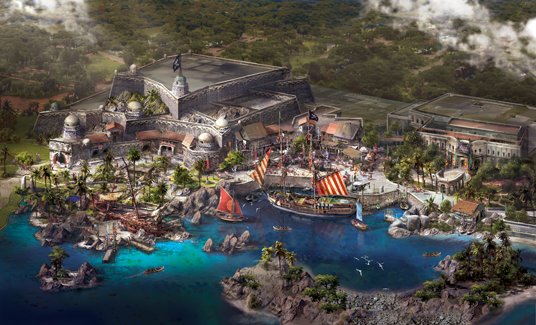This detailed illustration depicts a scenic, island-like village or private harbor, possibly representing a significant historical or fictional property. The aerial view reveals a vibrant port surrounded by lush tree lines, scattered clouds, and magnificent palm trees. Dominating the scene are two substantial buildings, each adorned with flags and framed by gigantic rocks that form a singular entryway into the harbor. 

The harbor itself hosts several ships and boats, varying in size and features. A substantial ship, docked in the harbor, is seen lowering its red and white striped sails. Nearby, a smaller vessel sails with blue sails, while another small boat features striking red sails. A distinct long wooden ship boasts yellow and white striped sails and flies a pirate flag.

The clear, aquamarine waters of the lagoon shimmer with lighter and darker shades, reflecting the sunlight cast on them. The buildings, made of gray stone with brown roofs, suggest an architecturally rich past, possibly resembling Roman or medieval styles. Amidst this setting, small, tree-covered islands dot the lagoon, enhancing the secluded and 'island-y' atmosphere of the property, which hints at being the luxurious compound of a very important figure or family.